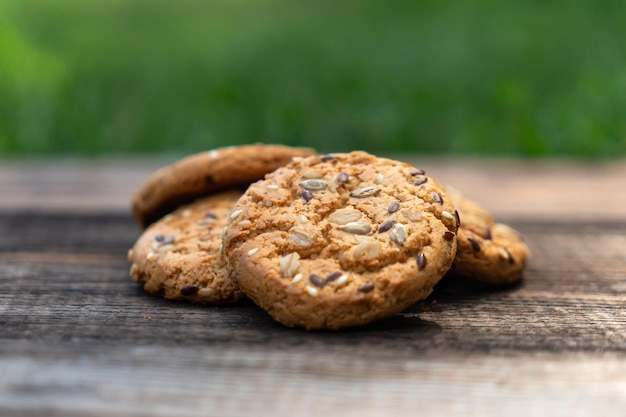In this image, a disorganized pile of four to six round cookies, predominantly brown in color, sits upon a wooden picnic table. The cookies appear to contain various seeds and grains, such as sunflower seeds, oats, and possibly other kernels. The table's surface is evident, and beyond it, the background features a blurred, bright green grassy area, indicating an outdoor setting. The photograph focuses closely on the cookies, highlighting their texture and seed-filled composition, reminiscent of standard cookies but distinguished by their unique ingredients.